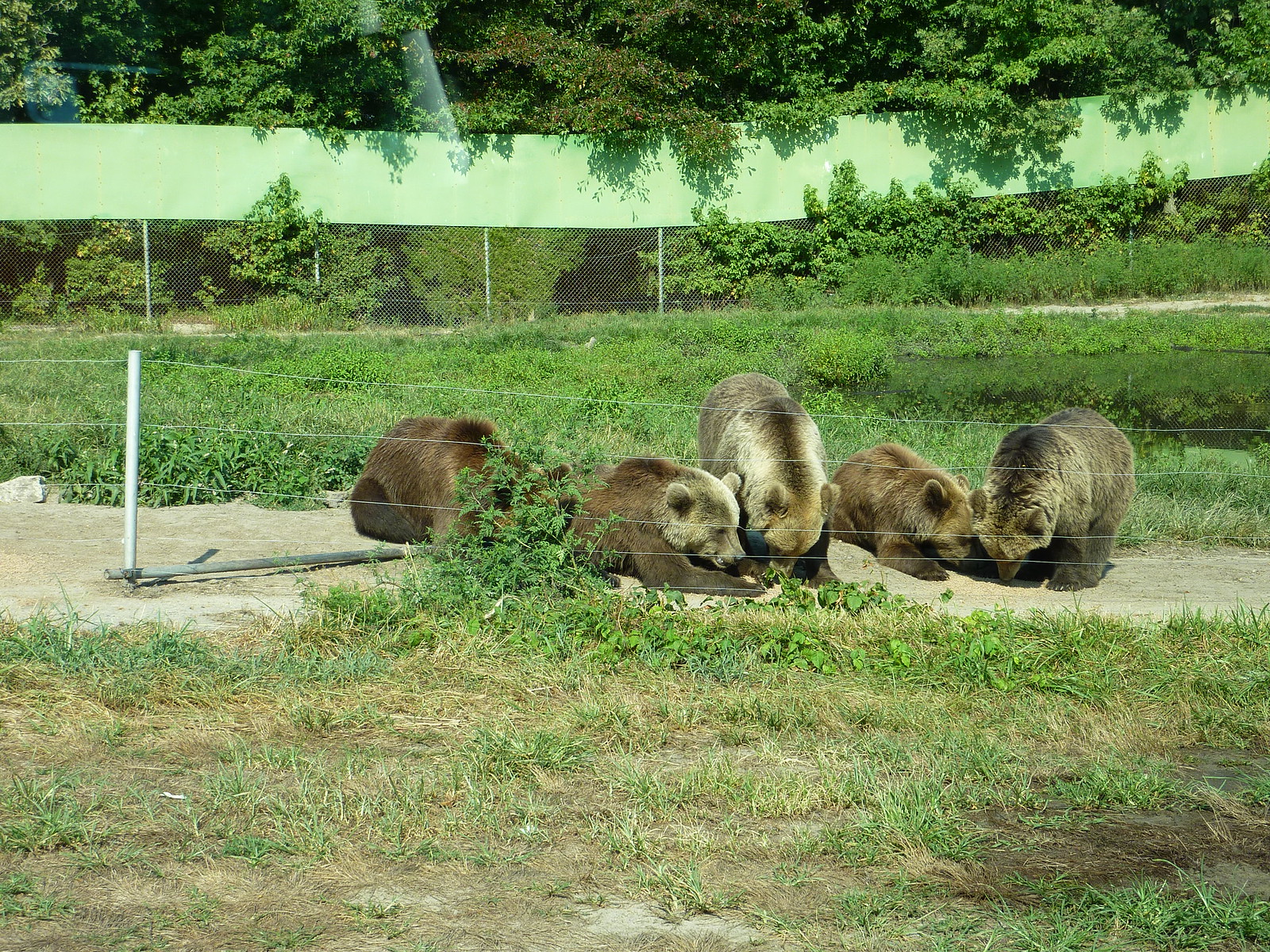The photograph captures five brown bears, appearing to be a mix of adult size and young adolescent cubs, within a fenced enclosure. They are positioned on a patch of dirt surrounded by patches of grass and tufts of taller weeds. The two leftmost bears are lying down, the middle one stands with its head lowered, the bear to the right of that is also lying down, and the rightmost bear is standing. The enclosure is secured by a metal wire fence with visible poles, and an additional whitish-greenish ceramic lining runs along the top to prevent climbing. Behind this fence is a green area painted or otherwise marked. In the distance, beyond the enclosure, trees and a forested area can be seen. The image includes a slight glare in the upper corner, suggesting that it was taken through glass. The foreground features a grassy area leading up to the enclosure.